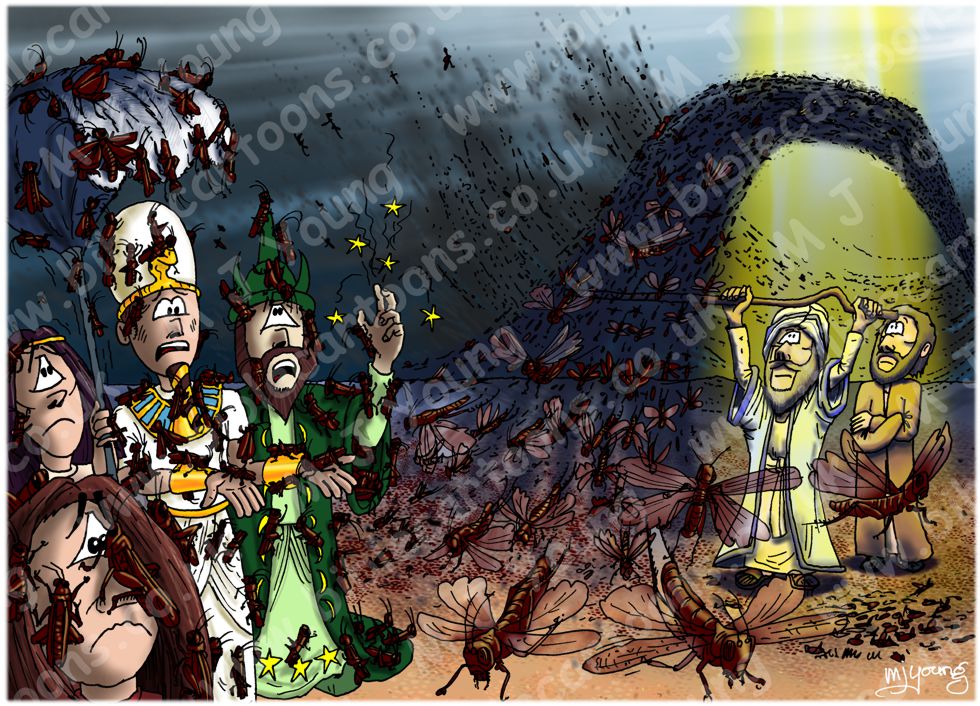This is a vibrant, Bible-themed cartoon watermarked with "Bill R. Cartoons" and "BibleCartoons.co.uk," featuring a plague of locusts swarming over biblical characters. The scene is bathed in light, possibly sunlight, breaking through a dense infestation of insects, adding a dramatic effect. The cartoon, reminiscent of 70s animation, showcases eight distinct figures: two on the left, panicking, and four on the right, including characters who appear to be a shepherd, a farmer, and individuals in Egyptian religious and royal attire. One of the figures on the right is throwing a staff into the sky in a dramatic gesture. Both the website and the creator’s signature, "T. Young," are visibly integrated into the image, with the website repeating several times from the left to the upper part of the image. The exaggerated, stylized eyes and horrified expressions of the characters capture the chaos and fear induced by the wave of locusts in this dynamic and detailed cartoon illustration.